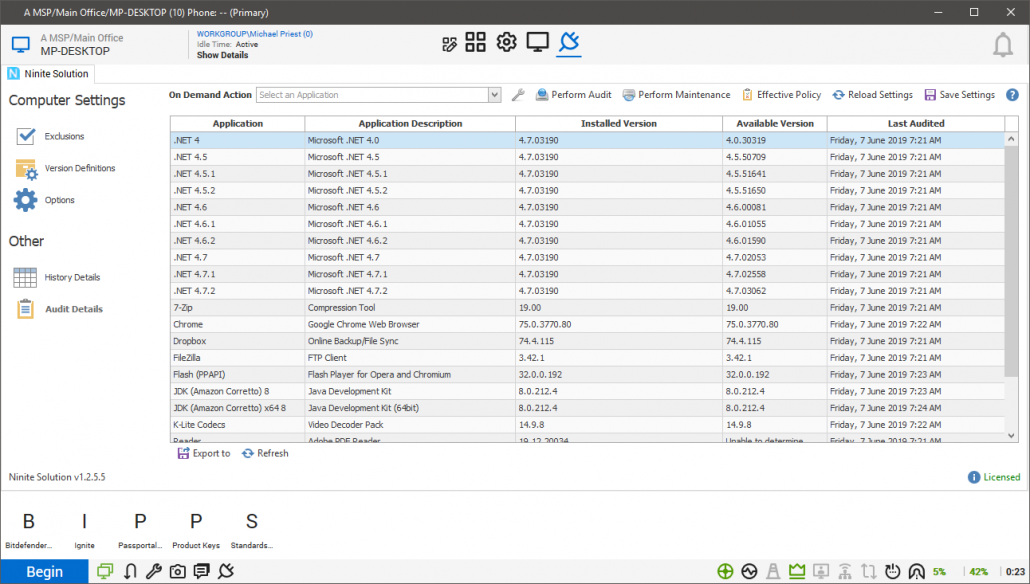This image depicts a computer screen displaying a program interface, specifically identified by a dark gray or black bar at the top that reads "AMSP / Main Office / MP Desktop 10 Phone Primary." A small blue icon representing a computer, labeled "MP Desktop," is also present in this bar. The display indicates the workgroup "Michael Priest 0" in blue text. 

Centrally located at the top middle of the screen, there are various small icons, including a settings icon, a computer icon, a plug-in icon, and a notification bell on the far right. On the left side of the screen, there are sidebar headings labeled "Computer Settings," encompassing options such as "Exclusions," "Version Definitions," and "Options," as well as an "Other" section with "History Details" and "Audit Details."

The main section of the interface reveals a detailed table listing several computer applications. Each row includes data such as the application name, description, installed version, available version, and the last audit date. At the bottom of the screen, there is an export function featuring a small purple 'save' button and a refresh button with two blue arrows. The section also includes a "Licensed" indicator on the right.

This detailed interface is part of a comprehensive system used for managing various applications and maintaining audit records on the computer.